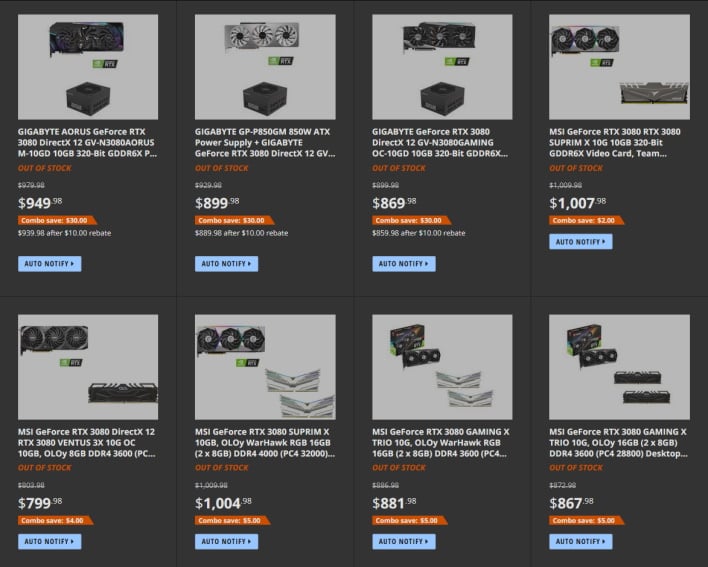The image displays a collection of eight power supplies and fans, with prices ranging from $799 to just over $1000. The first three items are from Gigabyte, while the remaining five are MSI GeForce products. Each product has a small, white image showcasing the power supply and its accompanying fan, accompanied by white text below detailing the product specifications. Notably, all items are currently out of stock, indicated by an orange "Out of Stock" label beneath each product. Despite being discounted for a combination deal where purchasing two products results in savings, none are available for purchase at this time. A blue "Auto Notify" button with black text is located below each item, allowing interested buyers to receive notifications when the products are back in stock. The entire image features a grey background with the eight product images overlaid.